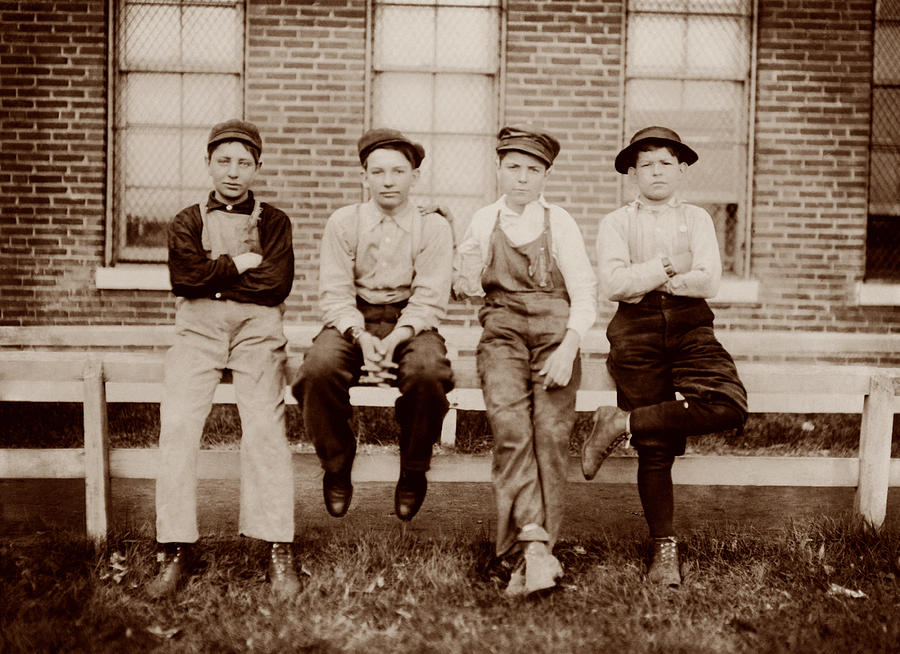In this evocative black-and-white photograph, four young boys are seated on a wooden railing in front of a well-worn vintage building. Each boy is dressed in overalls, and their hats add a touch of timeless charm. From left to right, the children are wearing distinctively colored pants: the first boy in white, the second in dark brown, the third in dark gray, and the fourth in dark brown. Three of the boys wear gentle, carefree smiles, while the boy on the far right gazes sternly at the camera, his expression markedly more serious.

The scene is framed by a patch of grass below, which exhibits a dark brown hue on the edges and a lighter gray shade at the center, illuminated by a soft light. In the background, a sturdy wooden fence stands as a barrier in front of an aged brick building with a couple of small windows, subtly hinting at the history and stories contained within its walls. The overall composition captures a nostalgic and poignant moment in time, reflecting both the innocence and varying moods of childhood.